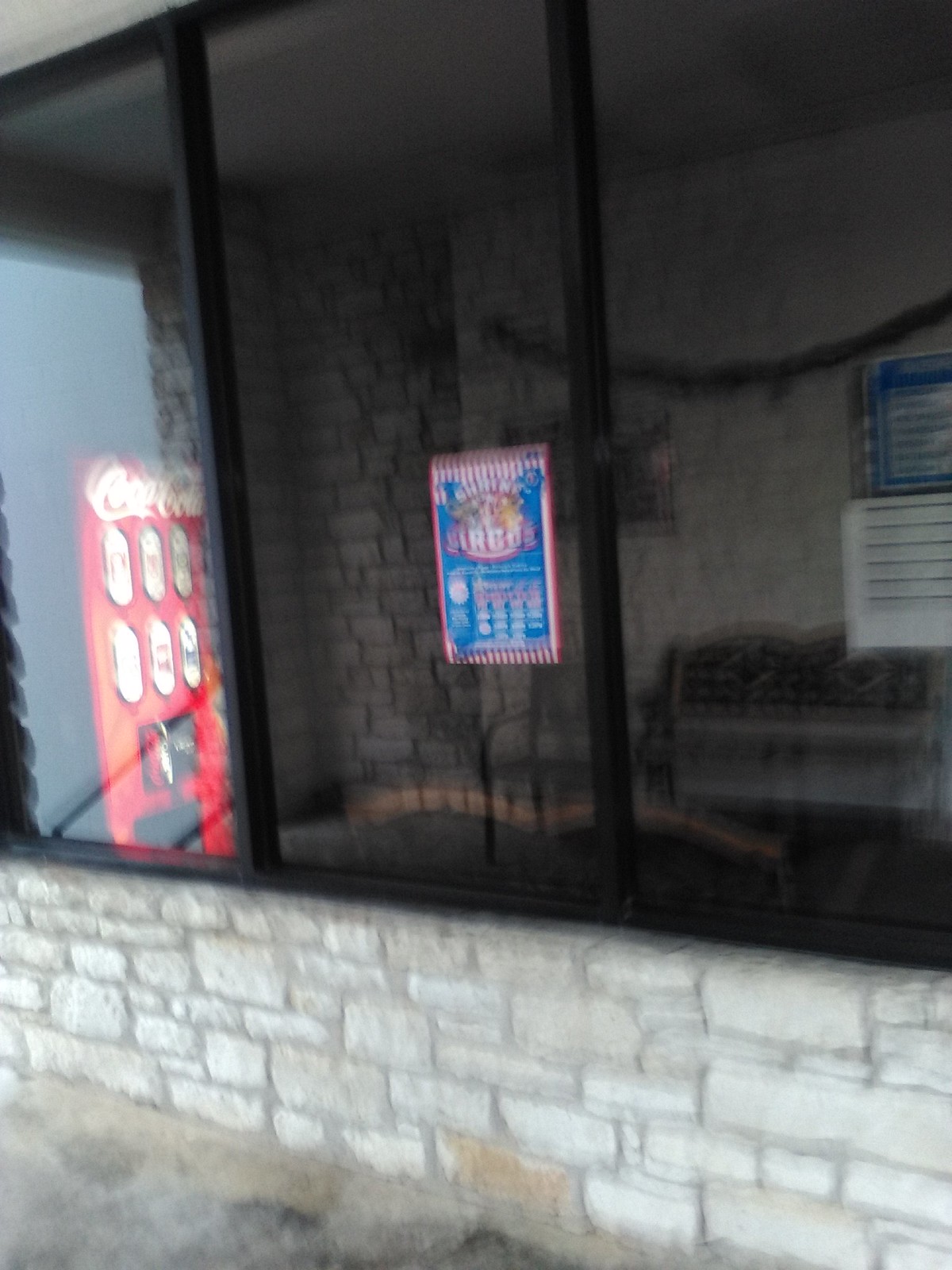This image, captured from the outside of a building, exhibits a slight blur and shakiness indicative of camera motion, perhaps due to a long shutter speed. The foreground features a short white cobblestone brick wall, rising only a couple of feet, before giving way to a large expanse of dark tinted windows. These windows are divided into three expansive panels. 

In the leftmost panel, a red Coca-Cola vending machine is discernible through the glass. The central panel offers a more obscured view of the interior, revealing primarily a circus poster affixed to an inside wall. The rightmost panel shows a faint glimpse of a bench within the room. The overall scene captures a moment of quotidian urban architecture, subtly animated by the blurred motion of the photograph.